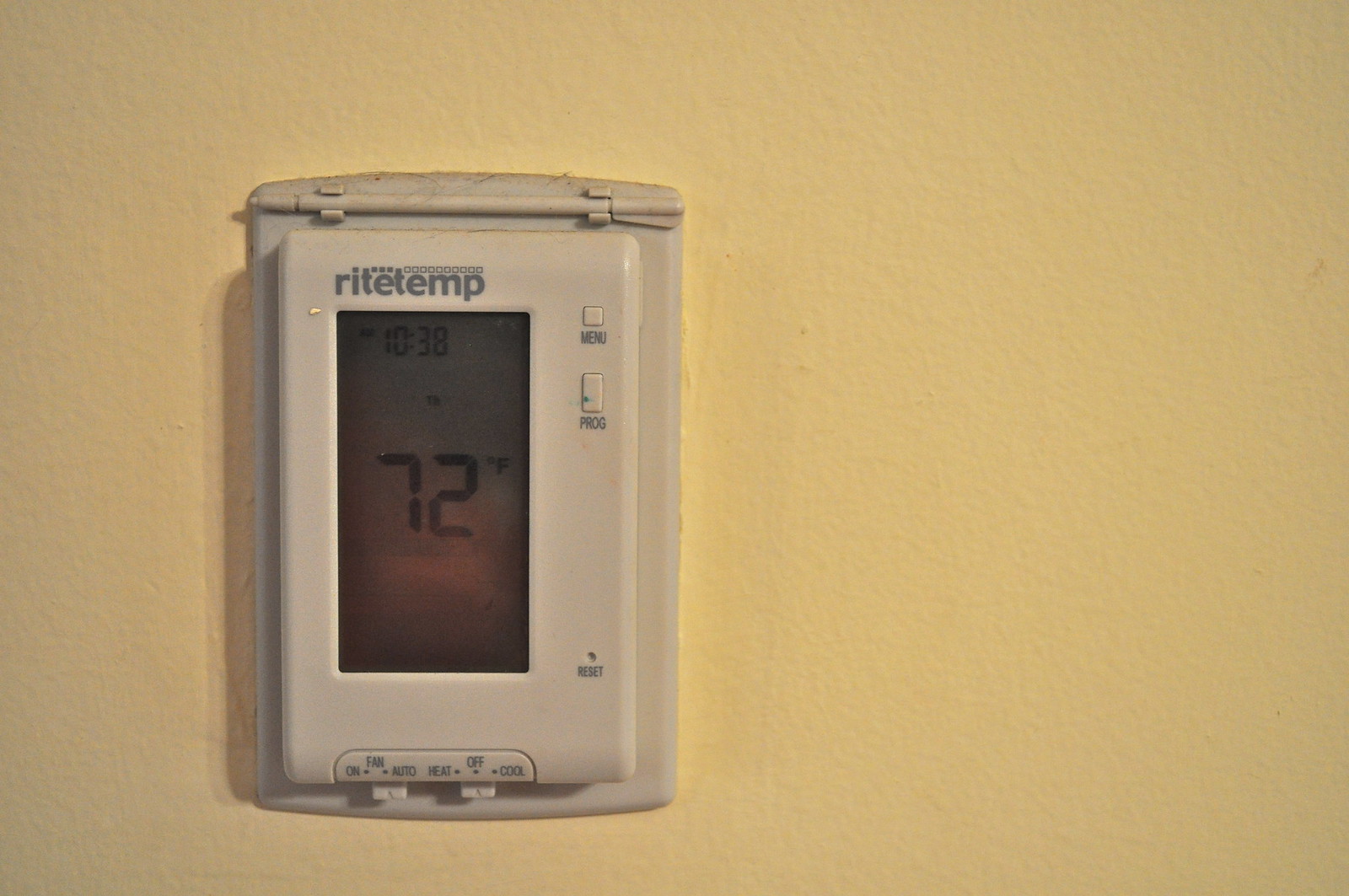This photograph captures a digital thermostat and an older air control thermostat mounted on a yellow-painted drywall. The wall features a muted, darker shade of yellow. Prominently centered is the vertical air control thermostat, which has evidently seen some years of use, as indicated by its somewhat dirty plastic rectangular casing. The digital screen in the center of the thermostat clearly displays the current time, 10:38, and the ambient temperature, 72 degrees Fahrenheit. Below the screen are two switches: the first switch allows you to toggle the fan between 'On' and 'Automatic,' while the second switch offers options to adjust the system settings from 'Heat' to 'Off' to 'Cool.'